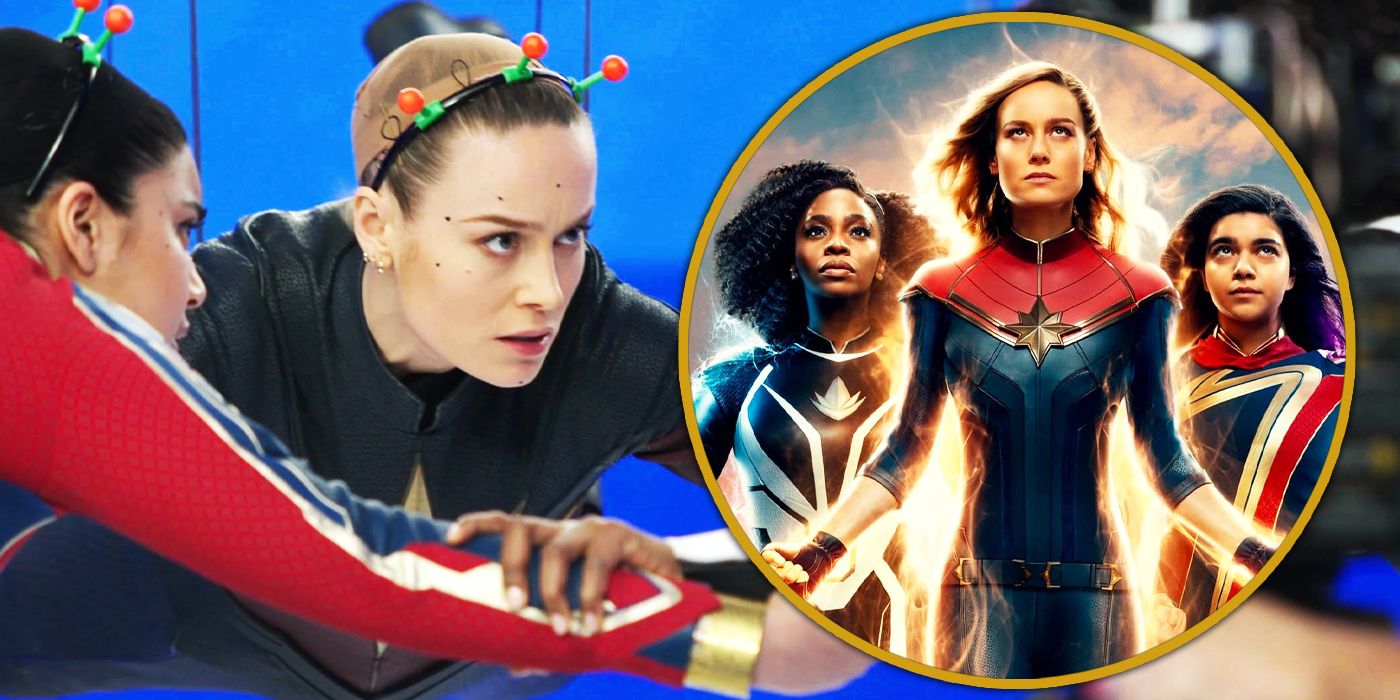The image captures a dynamic behind-the-scenes moment from the Marvel's movie, showcasing actresses Brie Larson and Iman Vellani in a setup prepared for an intensive CGI shoot. On the left side, Larson (Captain Marvel) and Vellani (Ms. Marvel) are seen wearing headbands with green markings and orange balls, likely for motion capture purposes. They stand in front of a blue screen, with faces adorned with tracking dots and wires attached to their outfits, suggesting they are preparing for a flying scene. To the right, the image transitions into promotional artwork featuring Captain Marvel, Photon (Monica Rambeau), and Ms. Marvel within a large gold-bordered circle. Each heroine, in costume, looks skyward with distinguishable energies; Captain Marvel glows with a yellow aura, Photon with blue, and Ms. Marvel with purple, all contributing to a powerful and visually striking poster-like composition.